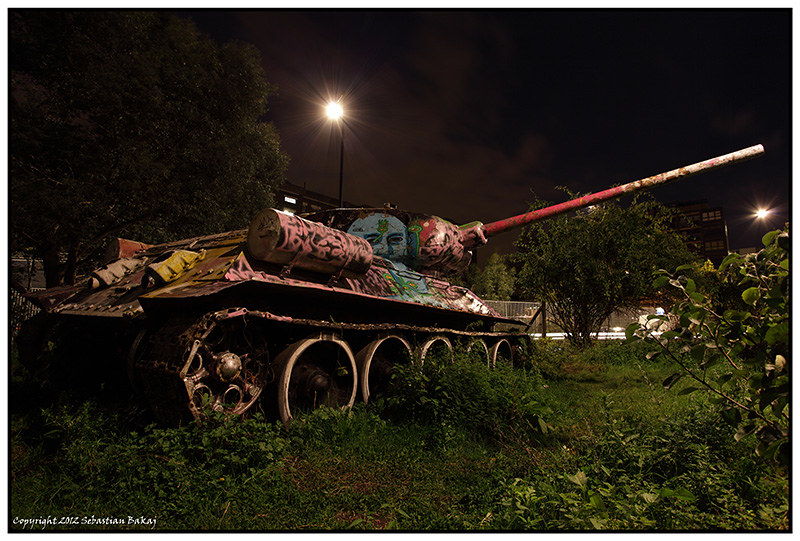This nighttime photograph captures a long-decommissioned, overgrown military tank, likely a Russian T-34 from World War II. The tank is vibrantly decorated with extensive graffiti: pink and reddish lines cover the barrel-like structure atop the tank, while the turret displays a partial blue face with quizzical eyes, accented by a green leaf on its forehead. The chin of this face extends down the body of the tank. The front of the tank is painted yellow, and the cannon features red paint with a white tip. Surrounded by thick vegetation and trees, the tank rests amid grass and weeds that have grown through its treads, indicating it has been stationary for an extended period. The scene is illuminated by streetlights, revealing residential or apartment buildings in the distance, adding an urban backdrop to this striking and colorful relic.